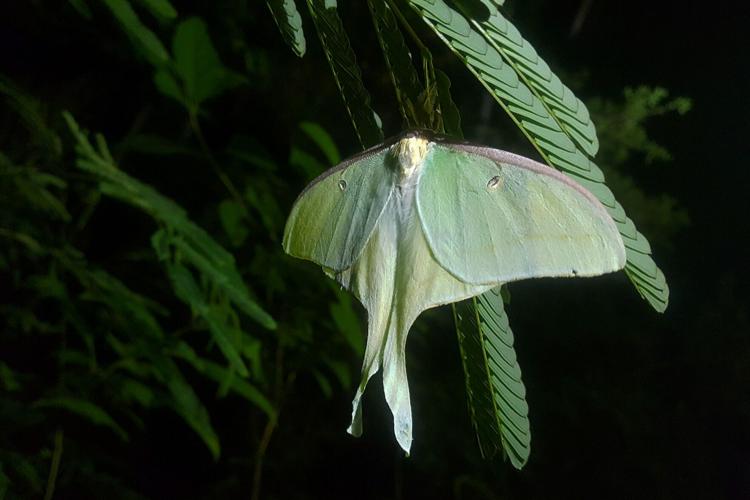This is a detailed close-up image of a luna moth, also known as the American moon moth, perched on a long, segmented green leaf. The moth is fairly large, its primary color being a vibrant lime green. The head of the moth is a whitish-yellow hue, and the body has a fluffy, almost yellow appearance. Its expansive wings are spread open, showcasing a pattern with distinct eye-like dots on each wing. The wings also possess vein-like structures and the front edges sport a faded purple color. The tail section of the moth is thin and splits into two trailing sections, resembling fish fins.

The background of the image is blurred, emphasizing the moth and the leaf it is resting on. This blurred background consists of dark greenery, suggesting the photo was taken in a tree-lined area, possibly at night, as indicated by the dark surroundings and the use of a camera flash. The lighting brings the foreground into sharp focus, capturing the intricate details of both the moth and the layered teardrop-shaped leaves that the moth blends seamlessly with. The overall scene presents a delicate and mesmerizing interplay between the insect and its natural habitat.